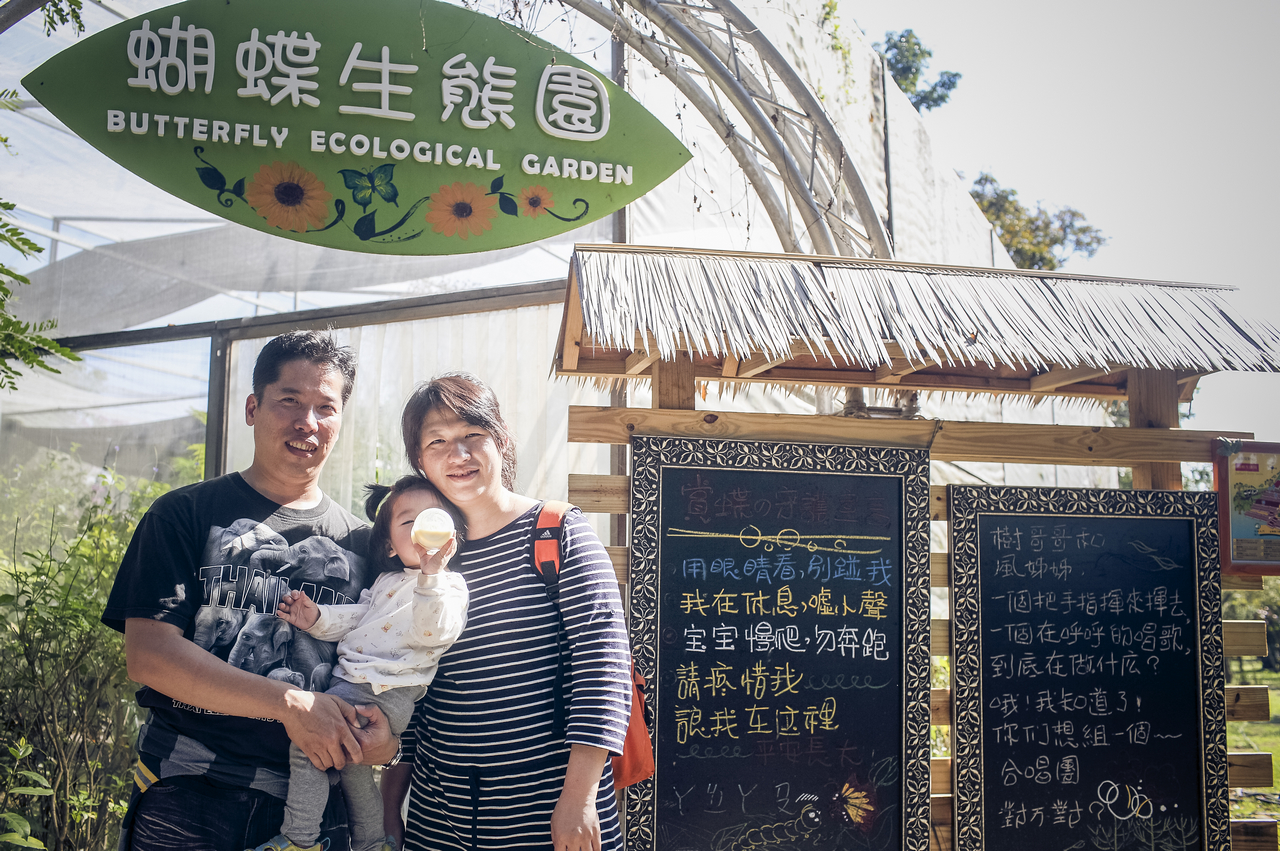This image captures a cheerful family moment at the Butterfly Ecological Garden, likely located in China, as suggested by the Chinese characters on the signs. The photograph, taken outdoors during the daytime in a rectangular frame, features a man, woman, and their toddler daughter of Asian descent. The father, positioned on the left, has short black hair and brown skin, and is wearing a short-sleeved black t-shirt featuring images of elephants and partially visible letters "T-H-I." He is holding his young daughter, who has her hair styled in pigtails and is captured drinking from a formula bottle, obscuring part of her face. She is dressed in a white shirt and grey pants, leaning back against her mother.

The mother, with her brown hair pulled back in a ponytail and brown bangs, is dressed in a black and white horizontal striped dress with long sleeves. She has an orange backpack, likely Adidas, slung over one shoulder. The family is positioned in front of an enclosure adorned with plants and mesh netting, indicating the butterfly garden behind them. Above them, a green leaf-shaped sign prominently displays the words "Butterfly Ecological Garden" in white print. To their right, a wooden stand with a thatched roof displays chalkboards inscribed with Chinese characters. The bright yet gray-hued sky forms the backdrop of this serene and intimate family photograph.